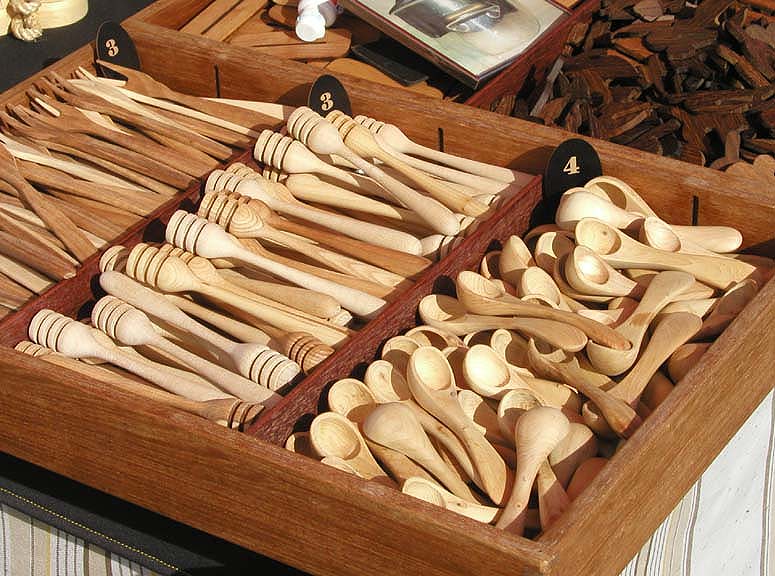This is a detailed photograph depicting a variety of wooden kitchen utensils organized in a dark, reddish-brown wooden box with three compartments. In the front section, several deep wooden spoons with thick handles, akin to those used for Epsom or lavender salts, are arranged neatly. These spoons resemble Chinese soup spoons and are clustered next to a black oval tag displaying the number "4." The middle compartment features wooden honey stirrers, designed with a combed cylindrical end and ridges, sitting beside a label marked with the number "3." In the rear section, small wooden forks with two tines are visible, also with a black tag indicating the number "3." Surrounding the wooden container are other indistinct items, including what seems to be a picture frame. The utensils rest on a white cloth adorned with beige and peach lines, and there is no text present to further describe the objects.